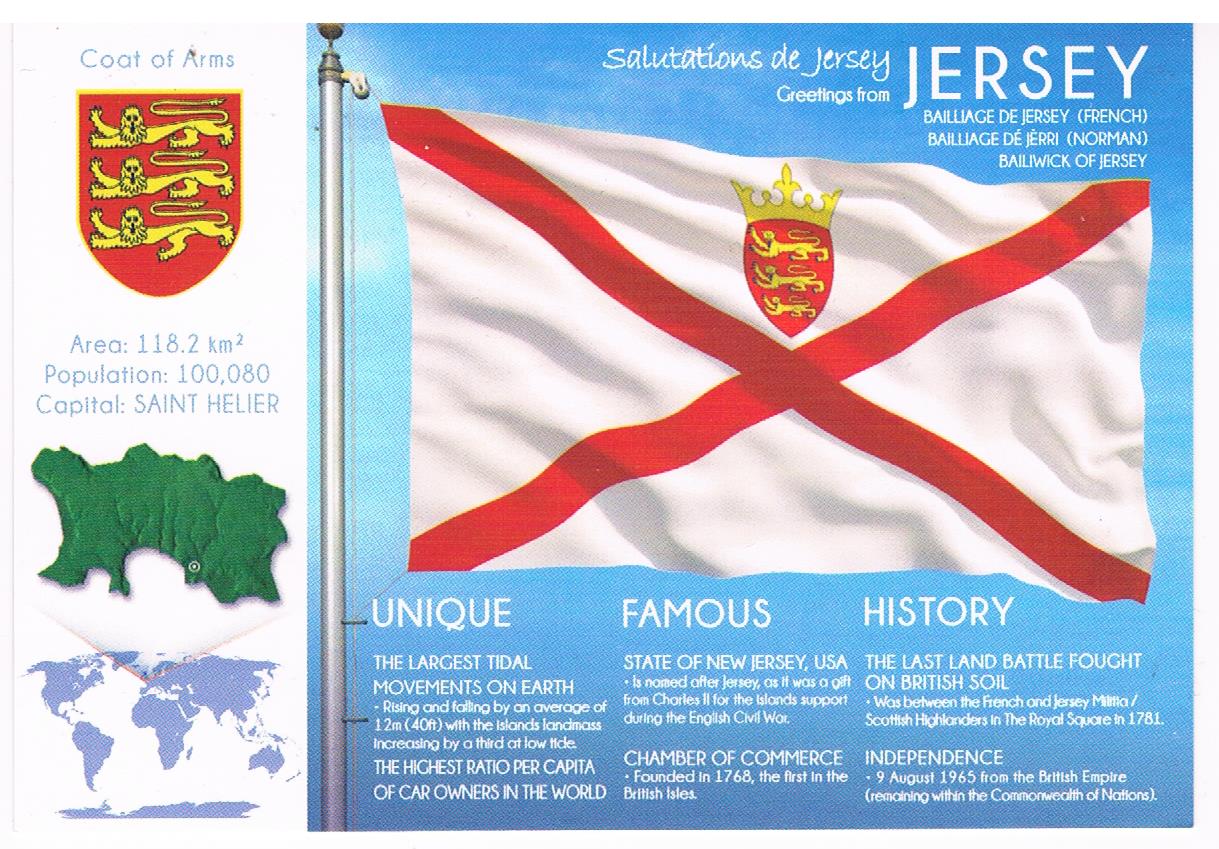The image is an infographic for Jersey, featuring both visual and textual elements to provide an informative snapshot of the island. On the left-hand side, a vertical white bar runs the length of the infographic, displaying detailed information. At the top, there is a red and yellow coat of arms with three lions, followed by text listing Jersey's area as 118.2 square kilometers, its population as 100,080, and the capital city, St. Helier. Below this, a small green map pinpoints Jersey's location within Europe, accompanied by a world map for broader context.

On the right-hand side, the background features a blue sky against which a flag of Jersey is hoisted on a flagpole. The flag is characterized by its white field with a prominent red diagonal cross (forming an X) extending from corner to corner, and the same coat of arms at the intersection's top section. The top of this half of the graphic reads, "Salutations de Jersey," which translates to "Greetings from Jersey" in French, along with its equivalents in Norman ("Balayage de Jerry") and reference to the "Bailiwick of Jersey."

Towards the bottom, the infographic is divided into three columns labeled "UNIQUE," "FAMOUS," and "HISTORY." Under "UNIQUE," it highlights the largest tidal movements on earth. "FAMOUS" mentions the state of New Jersey, USA, which was named after Jersey. "HISTORY" notes the significance of Jersey as the site of the last land battle fought on British soil. Additionally, it states that the Chamber of Commerce was founded in 1768.